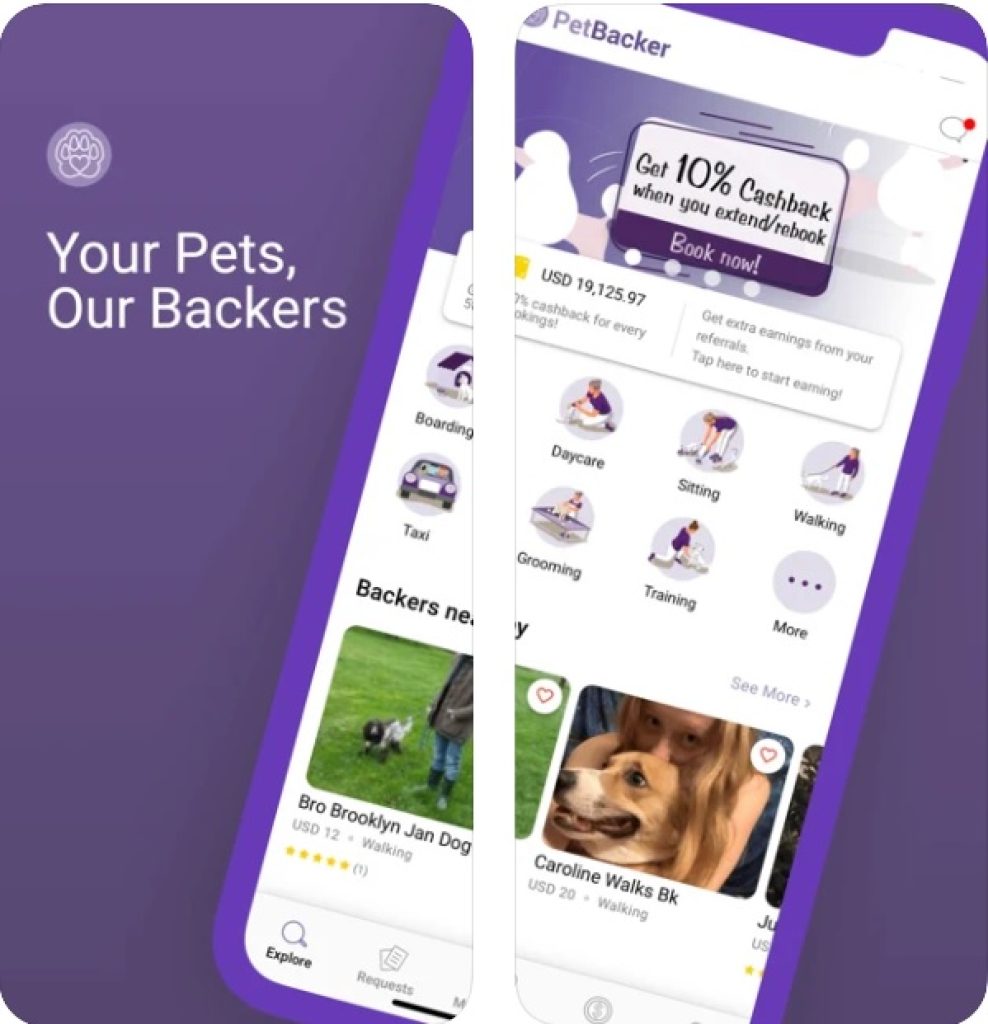This image features two screenshots of a mobile application, each displayed in the shape of a smartphone screen. 

**First Screenshot:**
- **Header:** "Your Pets, Our Backers" displayed in white text against a purple background with a circular paw icon.
- **Features Displayed:** The app offers various pet-related services such as boarding, taxi, daycare, sitting, walking, grooming, training, and more.
- **Visuals:** Icons representing different services are neatly arranged.

**Second Screenshot:**
- **Header:** "Pet Backer" with a promotional message, "Get 10% cash back when you extend/rebook," accompanied by a prominent purple "Book Now" button.
- **Info Section:** Details displayed include “USD $19,125.97” representing users’ total cash back earnings, with messages encouraging users to earn extra through referrals by tapping a specific link.
- **Service Listings:**
  - **Caroline Walks 8:** A walking service priced at USD $20, featuring an image of a dog with a person affectionately hugging its head.
  - **Bro Brooklyn Jan Dog:** A walking service priced at USD $12, depicted with a dog and a person walking. This service holds a 5-star rating based on one review.
- **Navigation Menu:** Options at the bottom of the screen such as "Explore," "Requests," and other typical app features.

Both images collectively emphasize the comprehensive pet care solutions and financial incentives offered by the app, illustrated through detailed visual elements and service options.